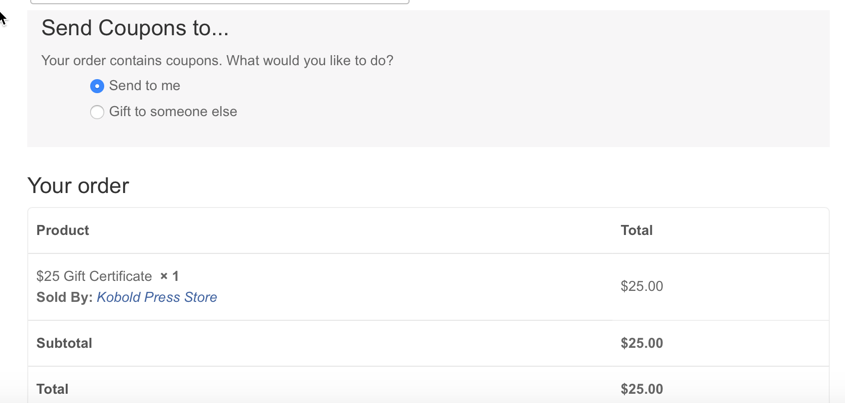The image displays a pop-up box associated with an order. The box has a grayish background with white areas for text. In the gray section, black text reads, "Send coupons to…," followed by, "Your order contains coupons. What would you like to do?" Below this, there are two options indicated by radio buttons: "Send to me" and "Gift to someone else." The "Send to me" option is selected, marked by a blue dot to its left.

In the white area below this, the text "Your Order" is prominently displayed in black. The section is divided into two columns: "Product" on the left and "Total" on the right. The product listed is a "$25 Gift Certificate," indicated as "x1" and sold by "Kobold Press Store," with "Kobold Press Store" appearing in blue text. The corresponding amount "$25" is listed to its right.

Beneath this, the subtotals are displayed. "Subtotal" and "Total" are both written in black text on the left, with "$25" shown in bold black text on the right for each.

In the top left corner of the image, the mouse cursor, depicted as a black arrow, is positioned next to the text "Send coupons to."